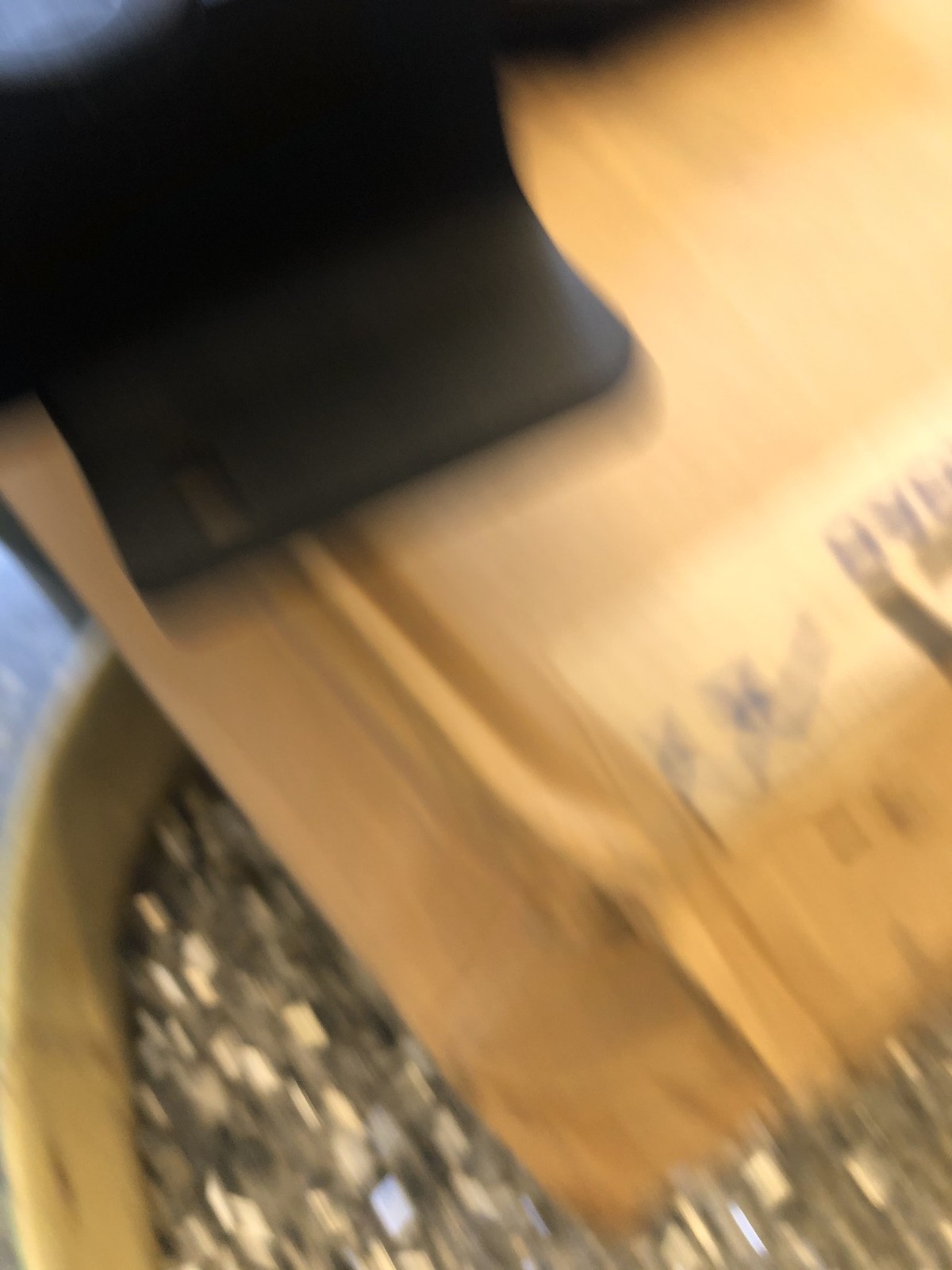In this blurry image, the bottom section showcases an expanse of loose gravel, characterized by its silvery hue interspersed with white specks, giving the appearance of numerous small rocks. This gravel seems to be contained within a large, concrete-like planter or vase. Resting atop the gravel is a sizeable manila envelope, distinguishable by a white postal sticker affixed to it. On top of this envelope lies a mysterious black device, whose exact purpose remains unclear. The overall scene suggests a juxtaposition of natural and man-made elements, captured with a slightly obscured clarity.